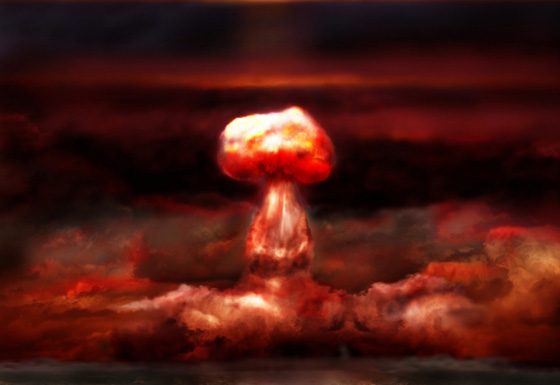The artwork depicts a dramatic bomb explosion, rendered in a realistic drawing style with a dark, somber palette of black, dark gray, and red. The sky is overwhelmingly dark, with heavy clouds in dark red and gray hues streaking across horizontally. At the center of the image, a towering, mushroom-shaped cloud bursts upward, its top portion the brightest element with vivid red and even a touch of yellow. The base of this cloud is a murky mix of black and muted red, creating a stark contrast against the dark sky. The scene is intense and pessimistic, capturing the devastating aftermath of a bomb, with no text or additional elements to detract from the powerful visual impact.